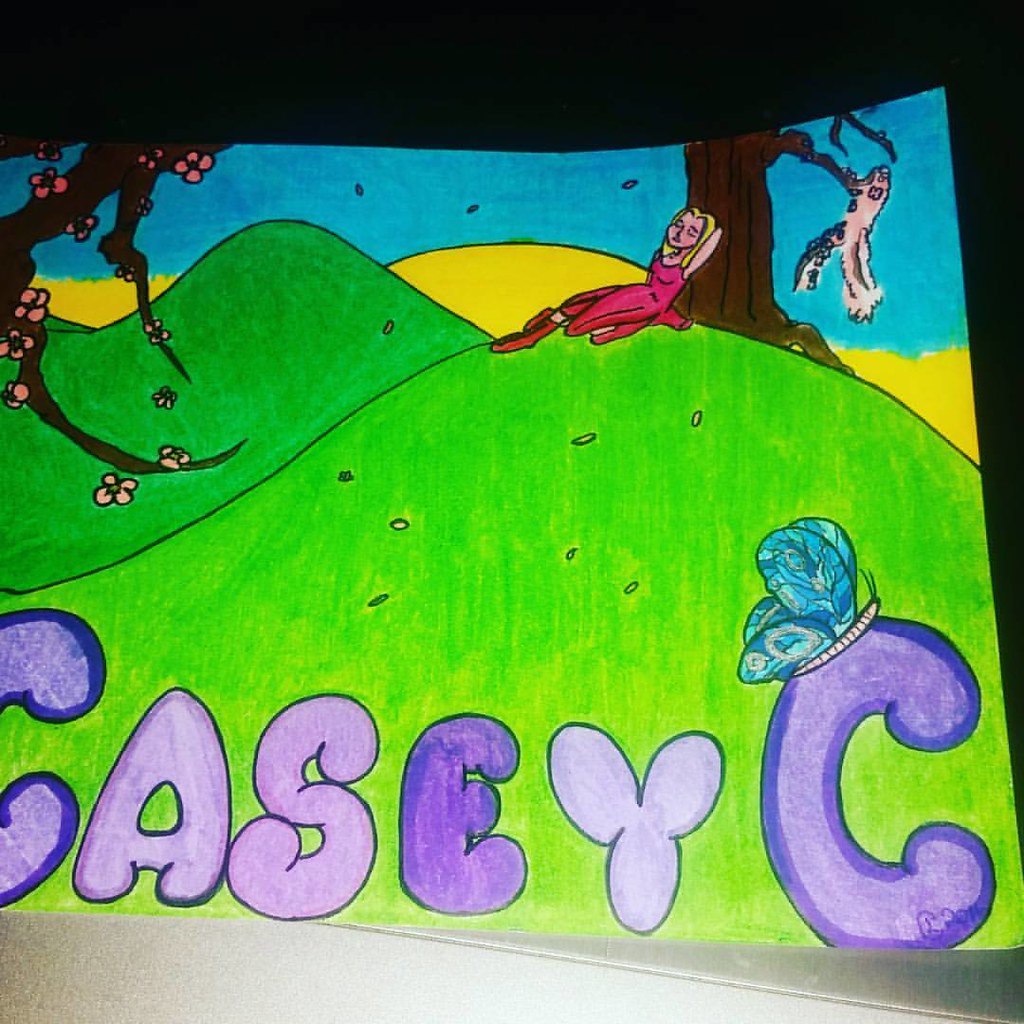A detailed caption for the drawing could be:

"This vibrant and whimsical drawing, potentially created by a young artist named Casey C., showcases an idyllic scene featuring a young girl in a hot pink dress lying against a tree on a grassy hill. The girl's blonde hair cascades gently as she leans comfortably, seemingly immersed in the tranquil surroundings. The artwork is signed 'Casey C.' in playful purple bubble letters, with a charming butterfly perched atop the second 'C,' adding a touch of animation to the signature. The background of the scene is adorned with blossoming trees, their branches dotted with delicate flowers whose petals drift gracefully through the air. A serene blue sky stretches above, hinting at the possibility of a setting sun that casts a warm glow over the landscape. The overall composition and attention to detail reflect a remarkable level of skill and creativity, making this piece a delightful and picturesque depiction of nature’s beauty."